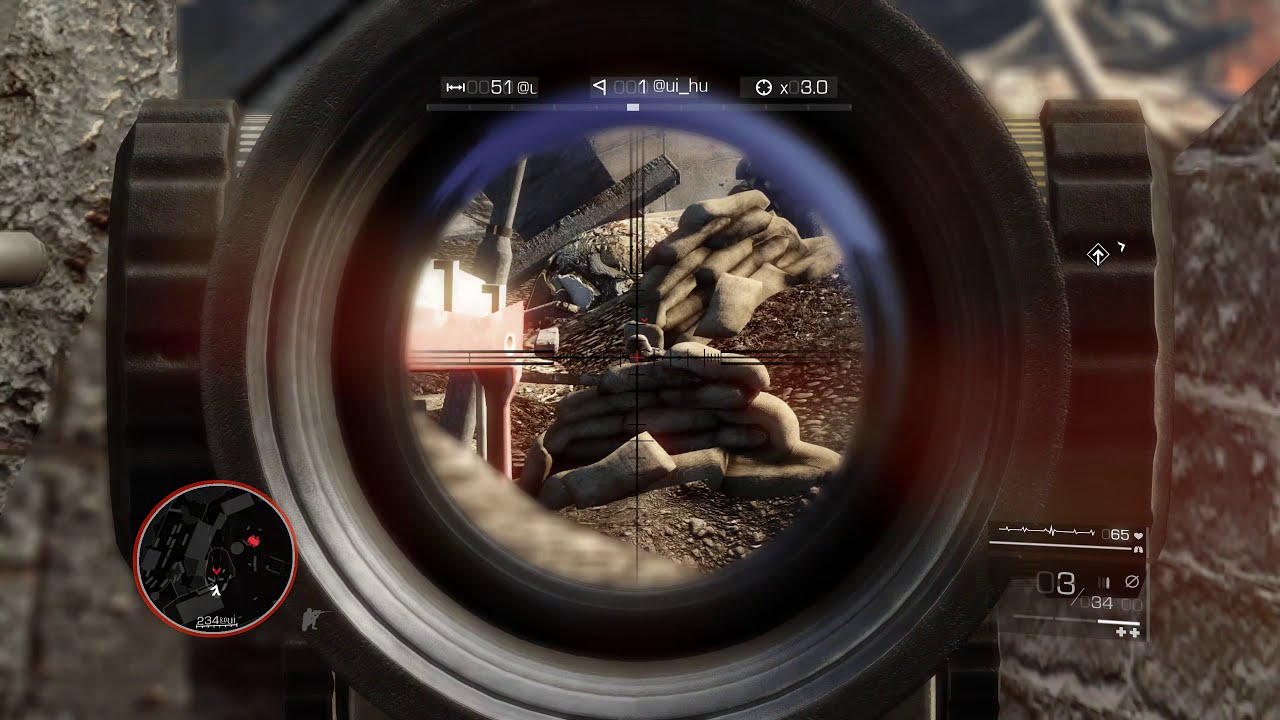The image depicts a first-person shooter video game, showcasing a sniper-like scope view. The scene through the scope reveals a jagged, rocky environment with debris, possibly remnants of buildings, and a lumpy, gray object resembling either rubble or a soldier’s head. A black crosshair marks the center of the lens, indicating a precise target. To the left, a radar and map are visible. Several UI elements are displayed: the top features "51" and "UI underscore HU," along with "3.0" indicating the zoom level. The bottom right of the screen shows ammunition details, "03/34," and a heart rate monitor reading "65." The left and right sides of the scope include gear-like adjusters, completing the immersive combat setting.